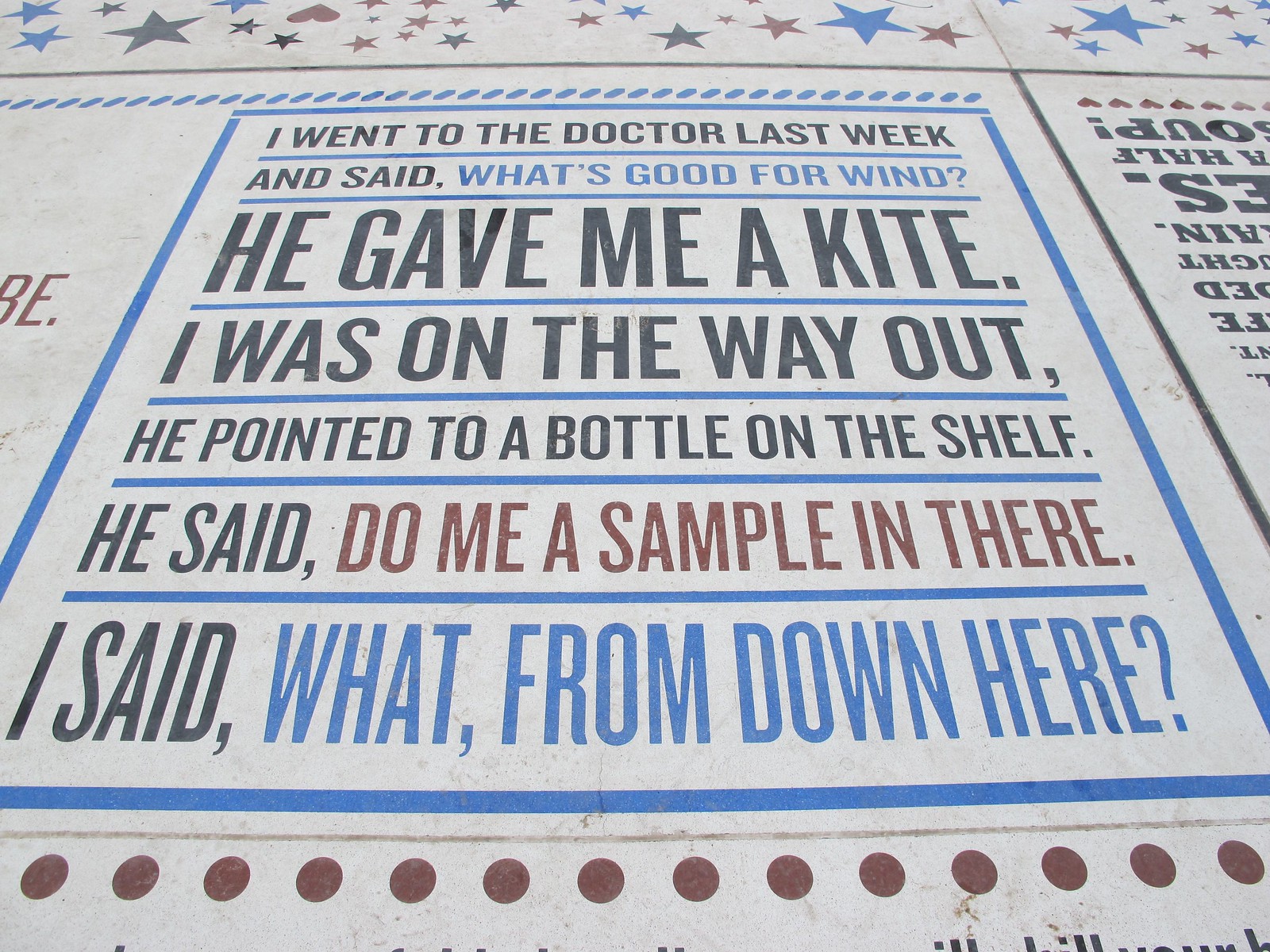The image is a color photograph of a humorous sign viewed from a slightly upward angle, revealing other partial signs with stars and a heart at the top edges. The sign itself is bordered in blue, featuring a comical narrative displayed in black, red, and blue text on a white background. At the top, black text reads, "I went to the doctor last week and said," followed by blue text stating, "what's good for wind?" In bold black text beneath, it humorously declares, "He gave me a kite." Below this, in smaller black text, it continues with, "I was on the way out," and, "he pointed to a bottle on the shelf." The punchline follows in black and red text, "He said, 'Do me a sample in there.' I said, 'What, from down here?'" Scattered at the bottom of the sign are several red dots, lining the border. The main focus of the image is this playful doctor-patient joke.